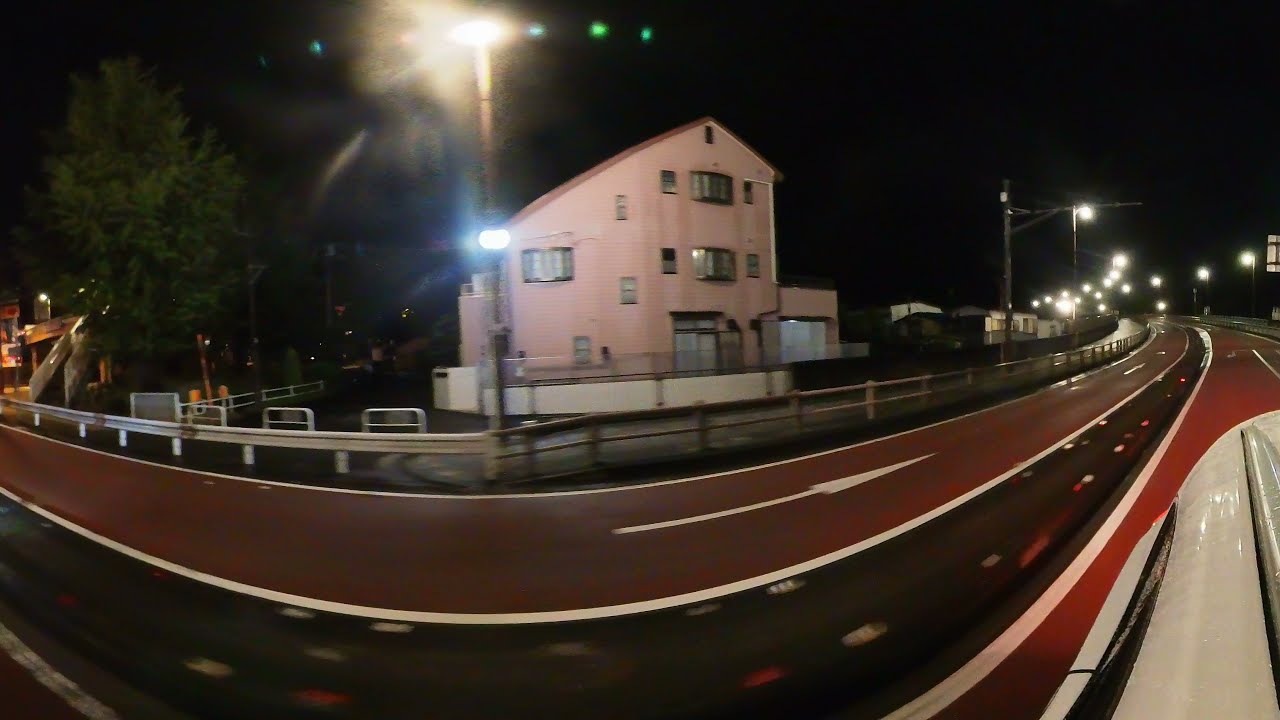This nighttime panoramic photograph captures a curved road scene with a wide-angle lens, emphasizing realism and photographic representationalism. The road, distinguished by its brown and black lanes, features white directional arrows, with a median separating the two directions of traffic. A white vehicle is visible in the bottom right corner, adding depth to the scene.

Dominating the center of the image is a pink stucco building, possibly a house or apartment, fronted by a large lantern and a significant light post. The backdrop of the night sky and the overall dark ambiance contrast with the various colors present, including shades of brown, black, white, red, beige, gray, and silver.

To the left, a silver guardrail outlines the road, shielding a building behind it, and another similar structure is seen farther along the right side. Additional streetlights and floodlights line the road, illuminating the path and contributing to the night setting.